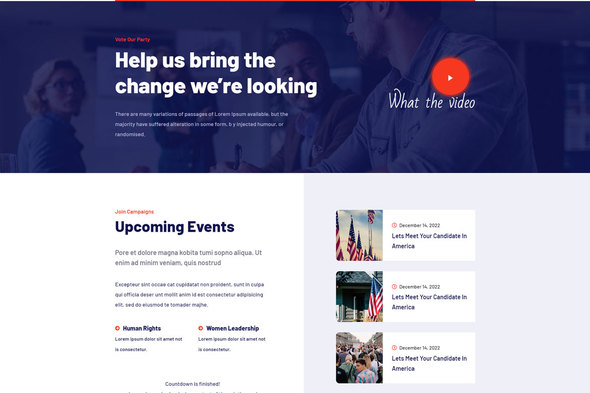This screen capture seems to be from a political campaign website. At the top of the image, there is a large navy box featuring a prominent message in orange and white text. The orange text is unclear, but the white text reads, "Help us bring the change we're looking for." Below this message, there are about two sentences in white text that are somewhat blurry, followed by the phrase "Watch the video" situated next to an orange circle with a white play button.

In the background, you can faintly see a woman with glasses and blonde hair, another person with crossed arms, and two men engaged in conversation—one of whom is holding a pen.

Scrolling down, there is text in red reading "Join campaign," followed by "Upcoming events" in navy. There is additional text that appears to be in Spanish. The section titles "Human Rights" and "Women Leadership" are rendered in navy, each accompanied by a red icon and a sentence in navy text.

Towards the bottom, there’s a segment titled "Countdown to something" with blue text.

On the right side of the image, there are a series of pictures:
1. An American flag set against a cloudy sky with the text "Let's meet your candidate in America," dated December 14, 2022, marked with a red icon.
2. An American flag outside a home with the same text and date, each accompanied by a red icon.
3. A crowd of people between two buildings also captioned "Let's meet your candidate in America."

These elements suggest a dynamic and patriotic campaign focused on community engagement and upcoming events.